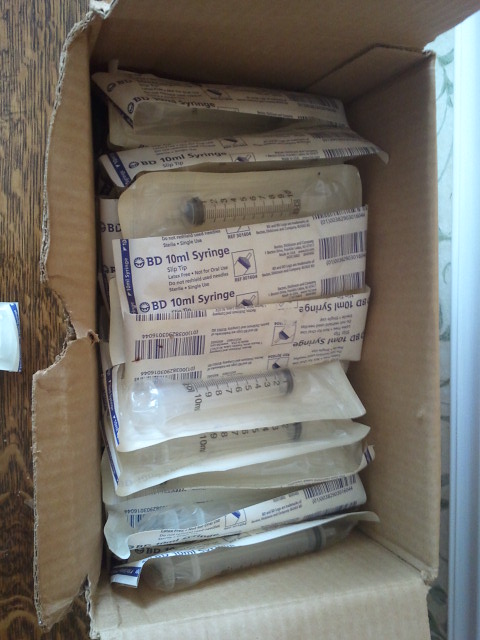The photograph captures a top-down view of a torn, opened cardboard box displaying its contents: multiple packaged BD 10 milliliter syringes. The box, brown and heavily damaged with a large chunk missing from its left side, sits on a tabletop made of dark wood on the left and a mixed dark and light brown floor on the right. Surrounding the box is a light blue wall with white molding visible in the background. Inside the box, the syringes are wrapped in clear plastic with blue and black text labels, barcodes, and small diagrams illustrating the syringe tips. The labels read "BD 10 milliliter syringe slip tip," indicating the type of syringes contained within. The photo has a glowing blue light illuminating the right side, adding an additional soft hue to the scene.